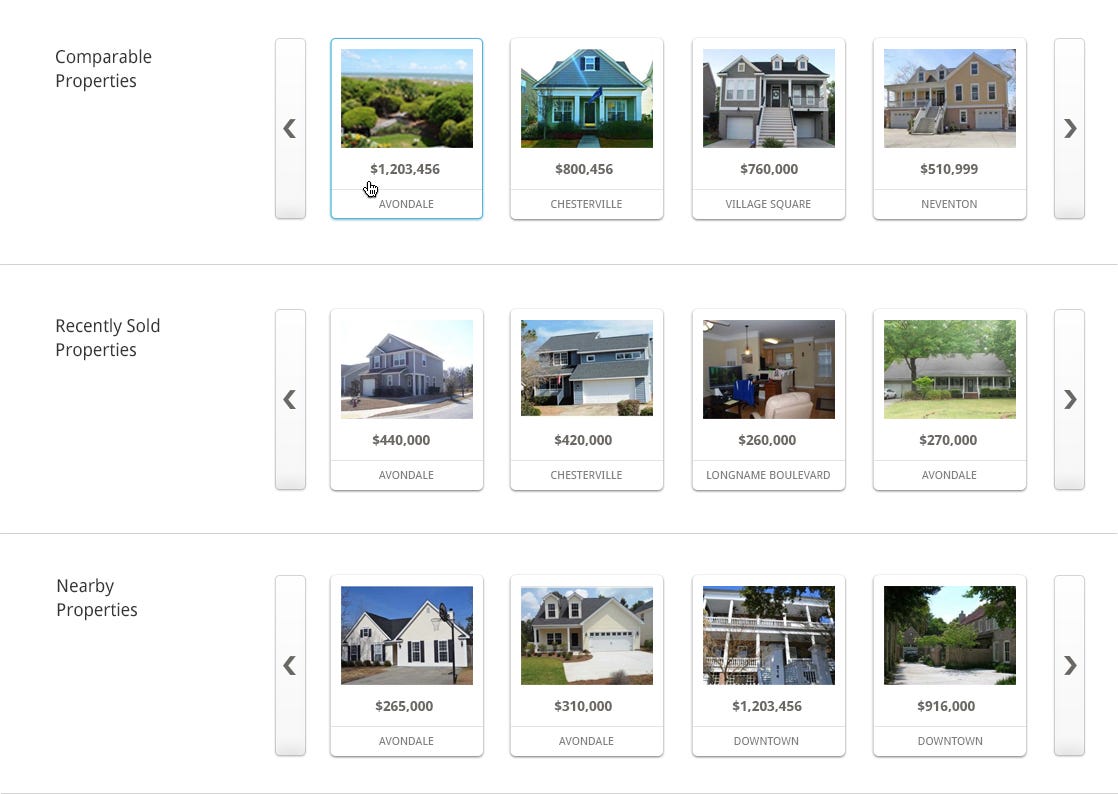**Detailed Caption:**

The image features a comparison chart with a white background, organized into three rows, each highlighting different categories of properties. 

- **Top Row: Comparable Properties**
  - The first property is listed at $1,203,456 and is located in Avondale.
  - The second property is priced at $800,456 and is situated in Chesterville.
  - The third property is valued at $760,000 and can be found in Village Square.
  - The fourth property costs $510,999 and is in Nevanton.

- **Middle Row: Recently Sold Properties**
  - The first recently sold property is from Avondale, sold for $440,000.
  - The second property, located in Chesterville, sold for $420,000.
  - The third recently sold property, situated on a long-named Boulevard, was sold for $260,000.
  - The fourth property from Avondale sold for $270,000.

- **Bottom Row: Nearby Properties**
  (This row wasn't explicitly described in the original text, so details cannot be provided.)

Each row and property is clearly labeled, offering a detailed comparison of property listings, recent sales, and nearby property values.